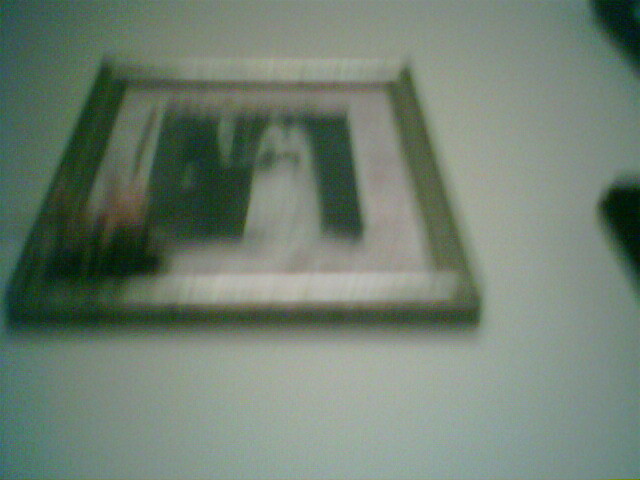The image depicts a very blurry photograph encased in a silver, shiny frame with a reflective finish, lying flat on a white surface. A small dark object peeks out from the right side of the surface, and a tiny black triangular corner is also visible on the right. The frame features a white mat and contains dried flowers in the lower left-hand corner, including one peachy-pink blossom with hints of green. Despite the blur, the photo inside is discernibly a wedding photo, likely in black and white. The bride is wearing a long white bridal gown, and the groom is dressed in a black tuxedo with a white shirt. Both their heads are not visible in the image.